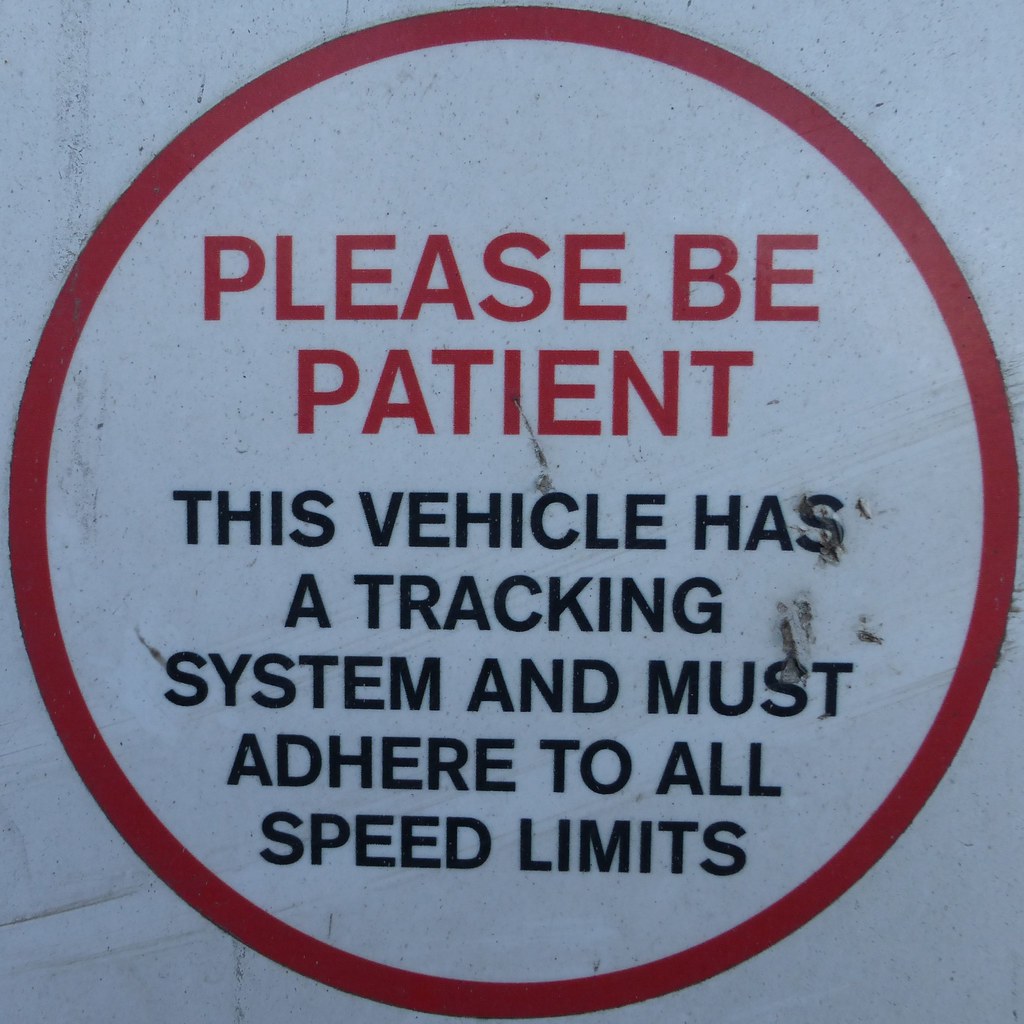The image depicts a close-up of a caution bumper sticker on a vehicle. The sticker consists of a red circle centered on a white square background, both of which show signs of wear and exposure to the elements, with scuffs and stains. Inside the red circle, the bold red text reads "PLEASE BE PATIENT," and directly below it, in black capital letters, the text states, "THIS VEHICLE HAS A TRACKING SYSTEM AND MUST ADHERE TO ALL SPEED LIMITS." This sticker is typically used on student driver cars or other vehicles where caution is advised.